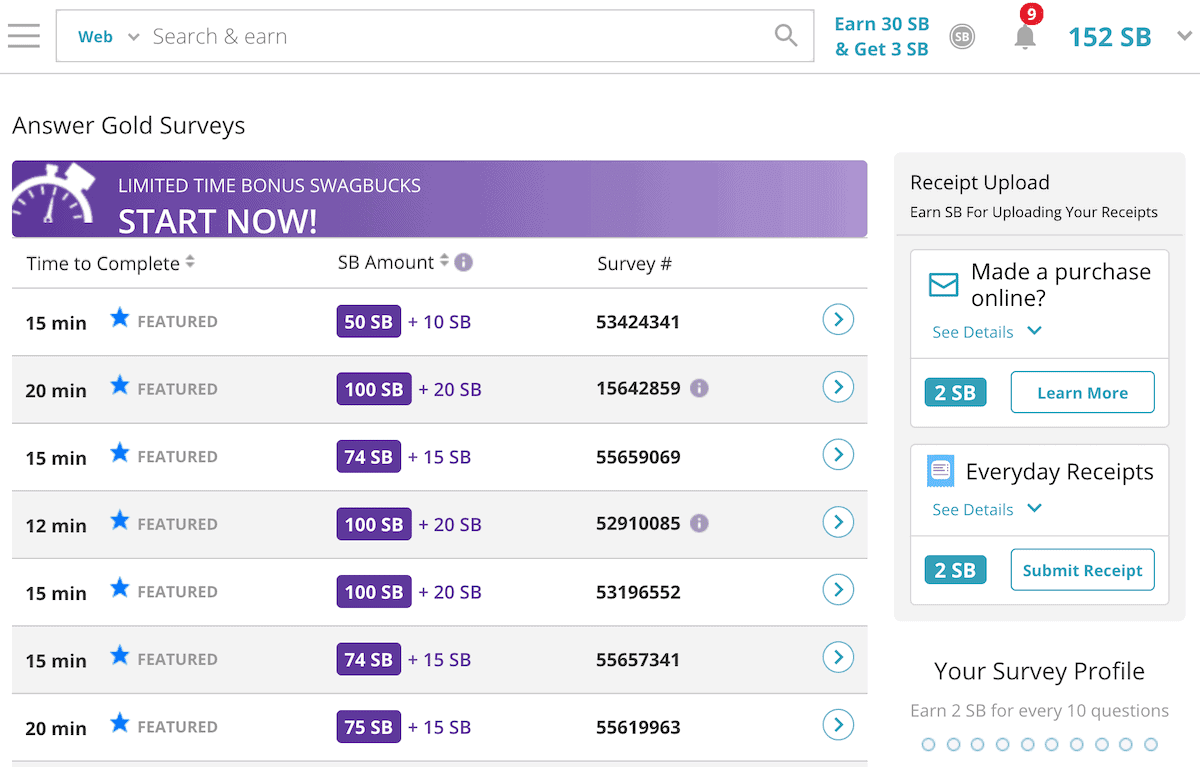This image is a detailed screenshot from a survey website, Answers Gold Surveys. At the top, a search bar is visible on the left for web searches, and to its right, there's an indication related to Swagbucks: "Earn 30 SB" and "Get 3 SB". A notification bell icon sits adjacent, bearing the number 9 in white on a red circle, highlighting pending notifications. The screenshot captures a balance of 152 SB accrued at that moment.

Directly beneath this is the main header, "Answer Gold Surveys". A prominent purple banner with white text reads, "Limited Time Bonus Swagbucks Start Now". Below this banner lies a list of available surveys. Each survey entry includes detailed information: the estimated time to complete the survey, a featured status indicated by a blue star if applicable, the Swagbucks (SB) reward for each survey, and its unique survey number. Each line item is equipped with an arrow button for easy navigation.

To the right of the survey listings, there is a section dedicated to receipt uploads titled, "Earn SB for Uploading Your Receipts if You Have Made a Purchase Online". This section includes a "See Details" link with an arrow and states that users can earn 2 SB with further details under "Learn More". Another box below this emphasizes "Everyday Receipts" with a similar "See Details", and states users can earn 2 SB by submitting a receipt.